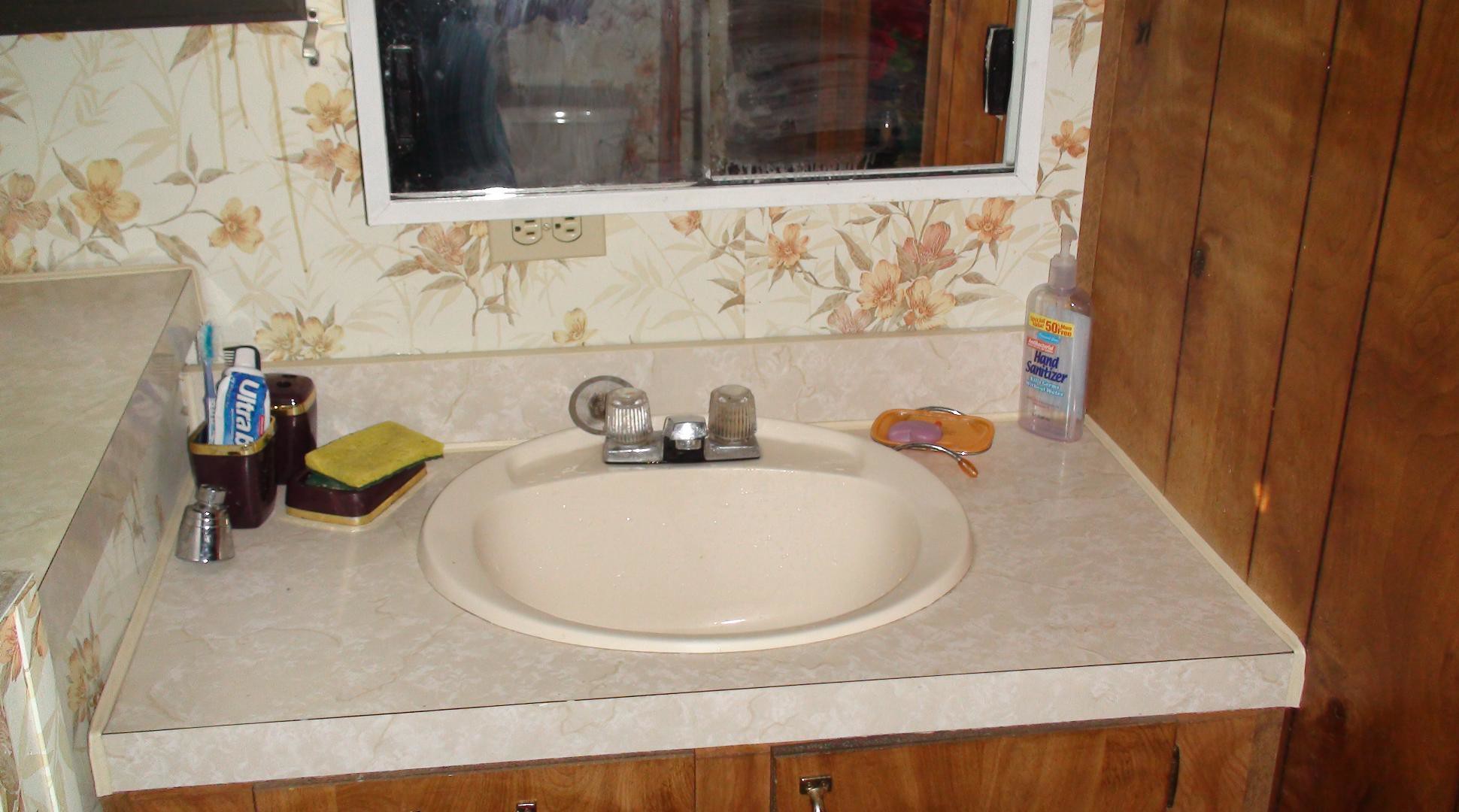This color photograph captures a vintage bathroom sink and countertop, reminiscent of the 1970s. The white porcelain sink features classic hot and cold knobs and a faucet characteristic of that era. The countertop is a light gray, nearly white, and bears signs of time's passage. 

On the right corner of the counter sits a clear bottle with a blue label and dark blue writing, its exact contents indiscernible due to its small size. In the left corner, two black cups reside; one of them holds a manual toothbrush and a partially visible tube of toothpaste with the recognizable "ultra" from the Ultra Brite brand, set against a blue background.

Above the sink, a mirror reflects part of the bathroom's interior. Within its frame, you can glimpse the top of a toilet on the opposite side and a portion of the wall. To the right of the sink, the wall is adorned with wood paneling, adding a warm, rustic texture to the scene. The back wall, supporting the mirror, displays wallpaper with a delicate floral pattern: light pink background interspersed with soft pink, orange, and yellow flowers, enhancing the bathroom's nostalgic ambiance.